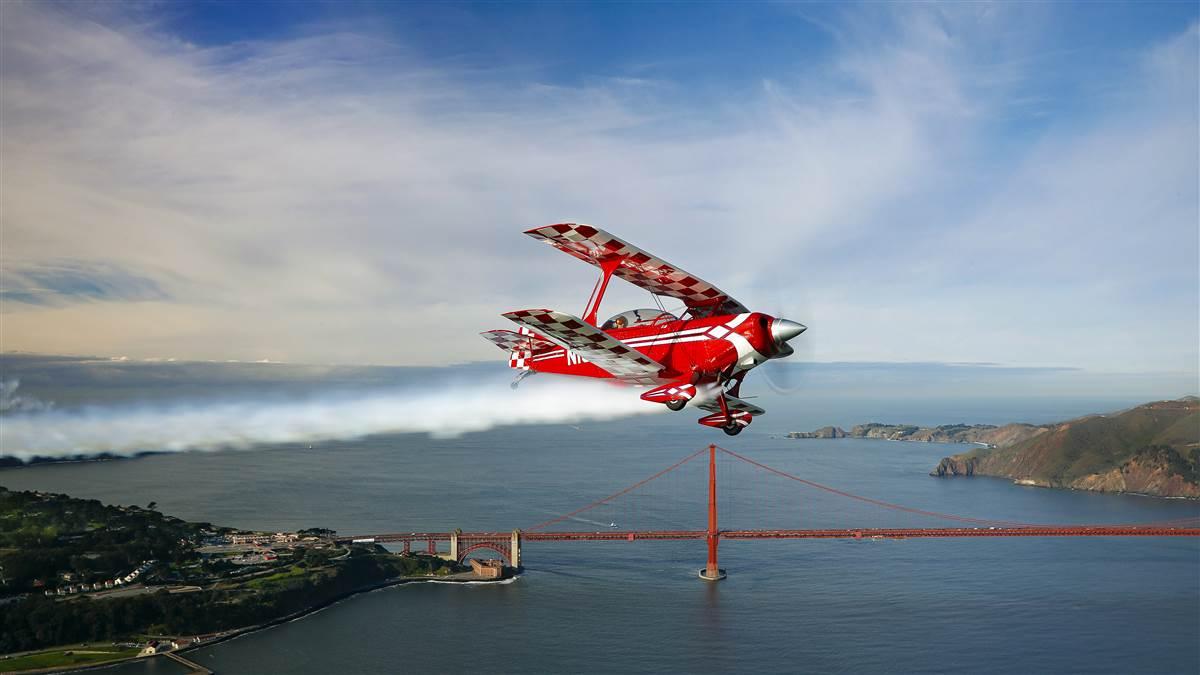The photograph, likely taken from several hundred feet in the air, offers a sweeping, daylight view of San Francisco Bay under a partly cloudy, blue sky. Dominating the foreground is a cherry red biplane with white striping and checkered details on the underside of its wings and tail, resembling the Purina logo. This classic stunt plane, with a silver propeller nose and a noticeable white smoke trail behind it, is flying to the right, slightly tilted to reveal its dual-wing configuration and single engine. Through its glass cockpit, a pilot is visible. Below the plane, the water of the bay reflects the expansive sky, while to the center and background, the iconic red spans of the Golden Gate Bridge stretch across the scene, connecting to the Presidio Park on the left. To the right, a small island, possibly Alcatraz, is discernible. The composition captures both the scenic and architectural landmarks of the bay area, framed by distant, hilly Northern California terrain.